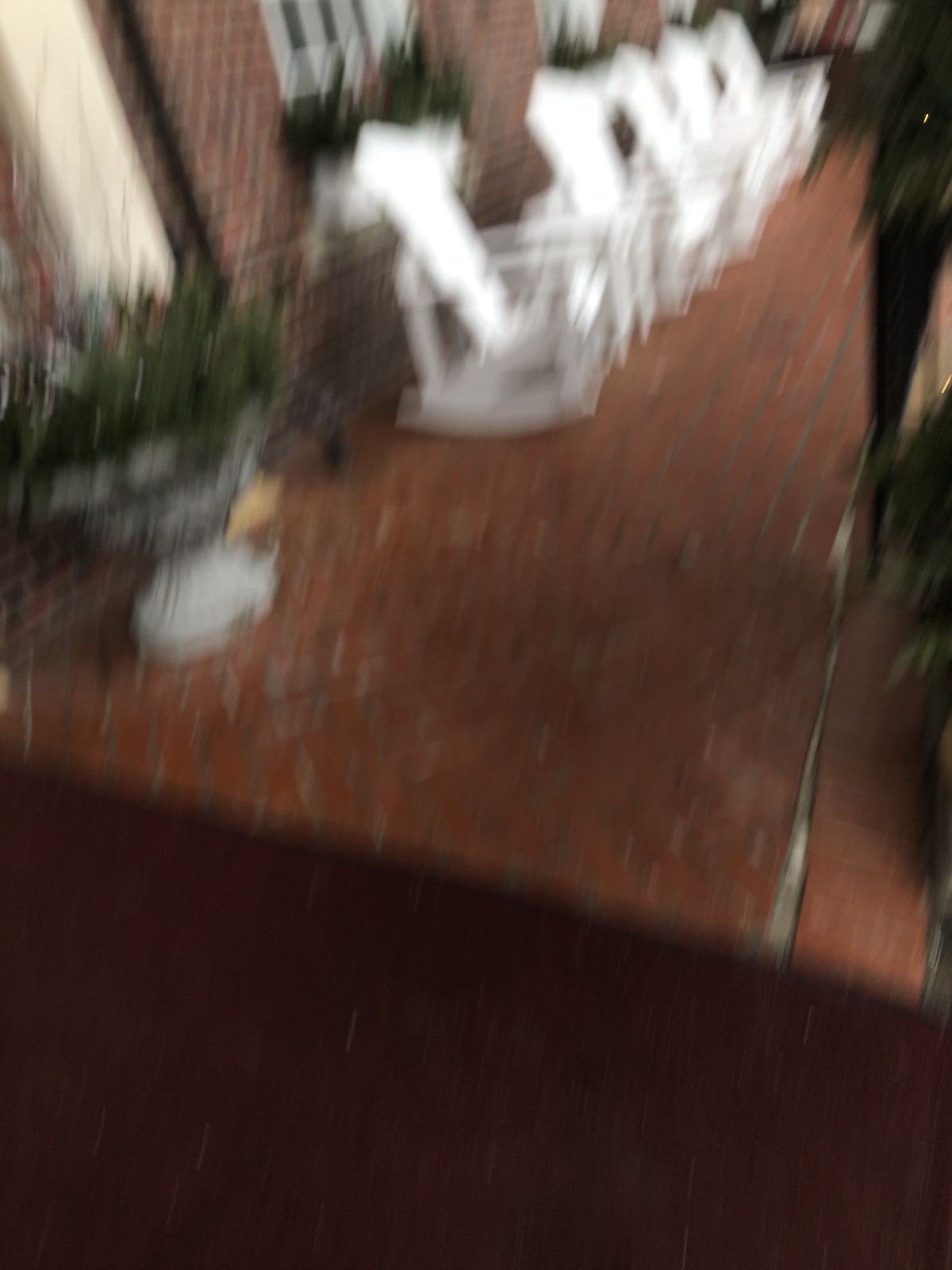This image is an extremely blurry photograph of the large front porch of a red brick home. The porch, which appears to be made of red bricks, features five white Adirondack rocking chairs lined up close to the front of the house. On the far left, a large gray stone planter holds greenery, though the exact type is indistinguishable due to the blurriness. The house itself, also constructed from red brick, has white-trimmed windows. Toward the right side of the photo, the outlines of the bricks are slightly more discernible. Additionally, there are steps leading up to the porch visible at the bottom of the photo. Shadows, possibly from the roof, cast across the scene, and the overall image is extremely jagged and out of focus, suggesting the photo was taken with an unsteady hand or under poor settings.